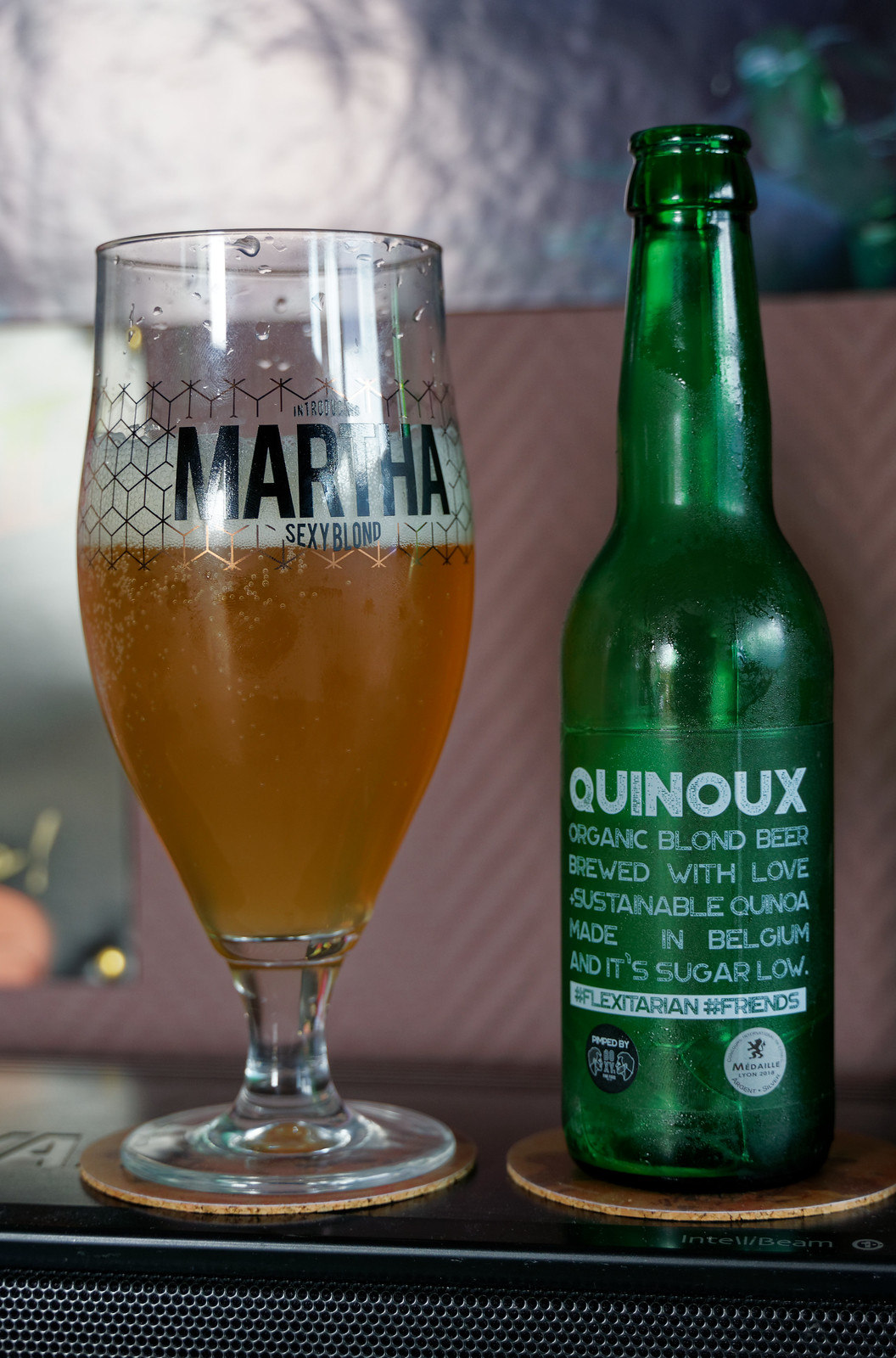The image features a green, standard-sized beer bottle and a tulip glass of beer, both placed on coasters atop a textured black surface. The bottle, which appears to be empty, prominently displays the name "Quinoux" in white letters, with the text below reading, "Organic Blonde Beer, brewed with love, sustainable quinoa, made in Belgium, and it's sugar low." This text is followed by the hashtags #flexitarian and #friends, alongside two emblems—one black with white lettering and the other white with dark lettering. To the left of the bottle is a tulip glass, about two-thirds full with beer, crowned with a light foam head. Imprinted on the glass are the words "Martha, Sexy Blonde." The background is blurred but shows a muted pinkish-brown wall and what appears to be a seated area, lending a cozy, intimate atmosphere to the setting.